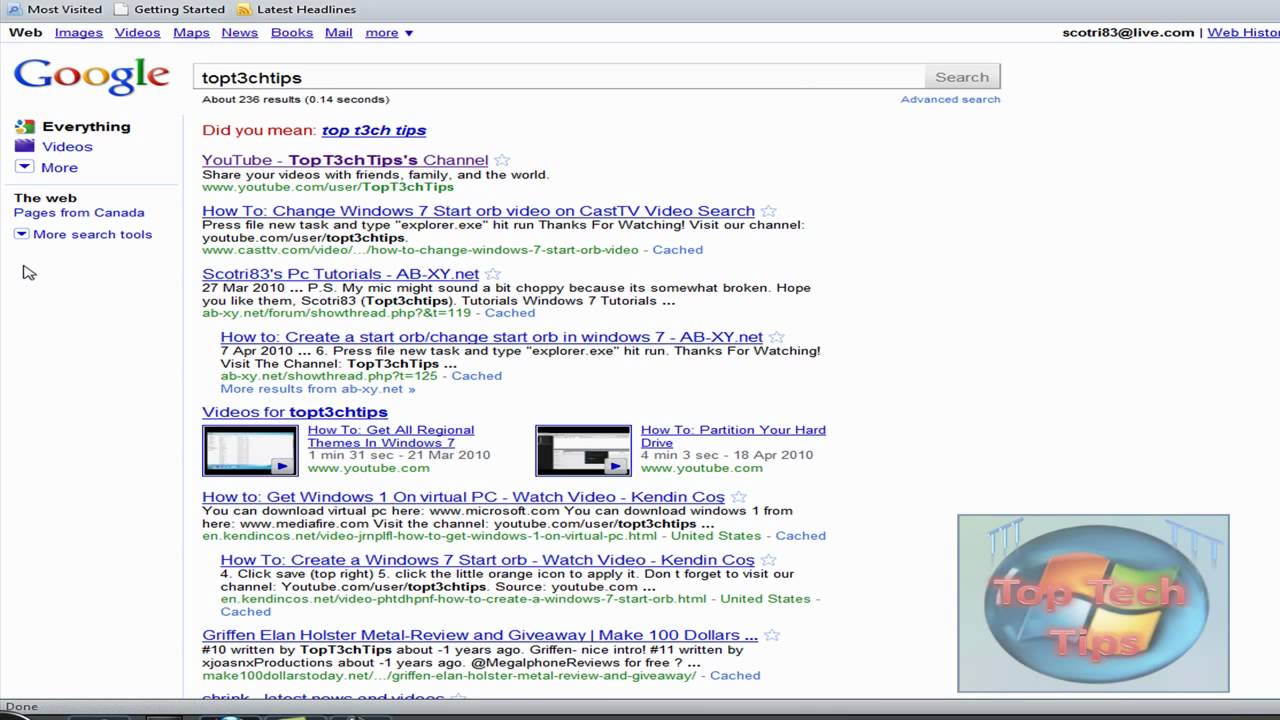This image displays a Google search results page. In the upper left corner, it lists categories including "Most Visited," "Getting Started," and "Latest Headlines." Below these are additional navigation options labeled "Web, Images, Videos, Maps, News, Books, Mail, More." The Google search bar shows the query "TOPT3CHTIPS" entered.

Below the search bar, the page notes "About 236 Results" and queries "Did you mean Top T3CH Tips?" The first search result is a link to a YouTube channel called "Top T3CH Tips," with the description "Share your videos with friends, family, and the world." This is followed by a tutorial result titled "How to Change Windows 7 Start or Video" from CastTV Video Search, explaining a procedure involving pressing 'File,' selecting 'New Task,' typing 'explorer.exe,' and hitting ‘Run.’ 

The next result is from a user named Scottree83, dated March 27, 2010, on ab-xy.net, featuring PC tutorials and a note about potential microphone issues. Another link shows a tutorial on "How to Create or Change a Start Orb in Windows 7," also from ab-xy.net.

Below these links are thumbnail images of two video results. The final search result listed is titled "How to Get Windows 1 on Virtual PC" by Kenton Cause.

Each entry provides brief descriptions and relevant details, making it easy to navigate through different tech tutorial resources and video guides related to the search query.